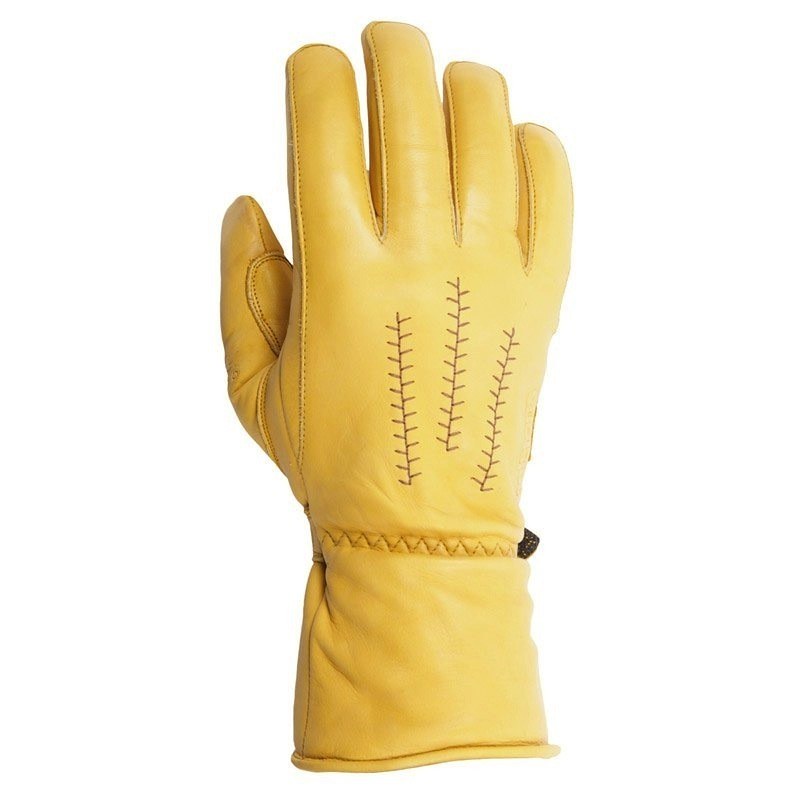The image showcases a sturdy yellow leather work glove, suitable for outdoor tasks such as ranching, chores, or gardening. The glove is prominently displayed against a plain white background with a light source coming from the right, casting subtle highlights. Crafted from thick leather, the glove features brown stitching along the fingers and thumb, which includes an additional padded area for extra durability. Distinctively, the glove displays three vertical designs on the back, each resembling a blade of grass or a head of wheat, with a central line flanked by shorter lines on both sides. The wrist area extends about three to four inches and has a zigzag brown stitching pattern, ending in a slightly rounded cuff. A small black tag is visible at the bottom right corner near the wrist, further detailing the handcrafted quality of the glove.